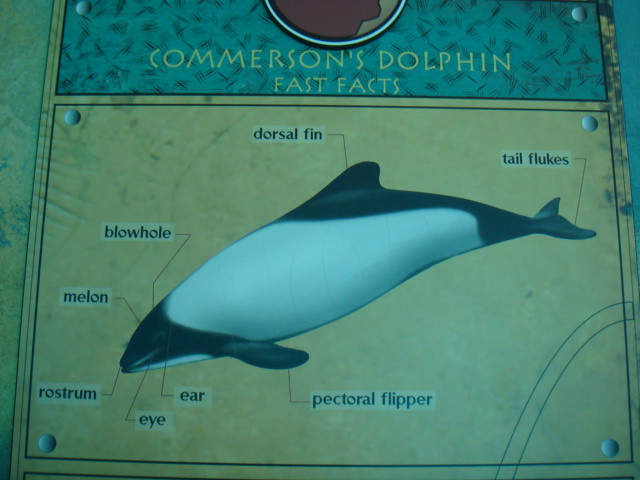The image showcases a detailed, rectangular illustration of Commerson's Dolphin, featuring "Commerson's Dolphin Fast Facts" in green text at the top. It appears to be some sort of educational plaque, possibly displayed on a website or in an aquarium. The dolphin, presented in profile, is identified by its distinctive black and white coloration: a black head, front flipper, dorsal fin, and tail flukes, contrasted by a predominantly white body. A yellow-colored background surrounds the dolphin's labels, with arrows pointing to various anatomical parts such as the dorsal fin, tail flukes, blowhole, melon, rostrum, eye, ear, and pectoral flipper. The corners of the plaque are secured with gray pins, adding to its display-like nature. The image includes a red and white logo at the top center, contributing to the educational presentation.